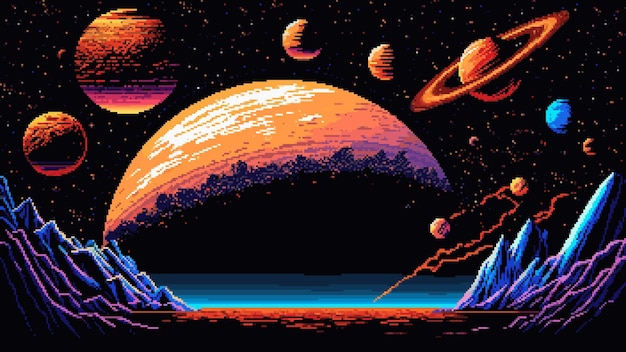The image is a highly detailed, digitally rendered illustration of an alien planet's landscape set in the vast expanse of space. The dark sky is peppered with stars, adding depth to the scene. Dominating the foreground, an enormous orange planet looms nearby, its silhouette hinting at a cityscape or terraform features. Surrounding this massive celestial body are several smaller planets, mostly orange in hue, and differing in size. Notably, a blue planet, resembling Earth, is situated on the right side of the image. The landscape underfoot features icy, cap-like structures and flat, orange terrain. To the sides, mountains and craters create a rugged contrast, some shaded in purple and blue. The overall style is distinctly science fiction, emphasizing the alien and fantastical elements of the scene.